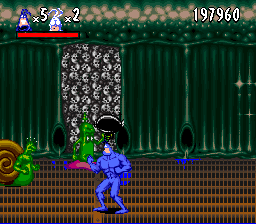A small, square image from a video game features a blue, muscular character with a white face striding across a pixelated grate floor. To the left, a giant snail monster looms menacingly. In the background, a slime monster slithers near two sewer pipes set against a green wall, both leaking blue liquid. The top left corner of the screen displays an indicator showing five lives left for the blue character and two lives for another character, accompanied by a health bar below. To the right, the score is prominently displayed.